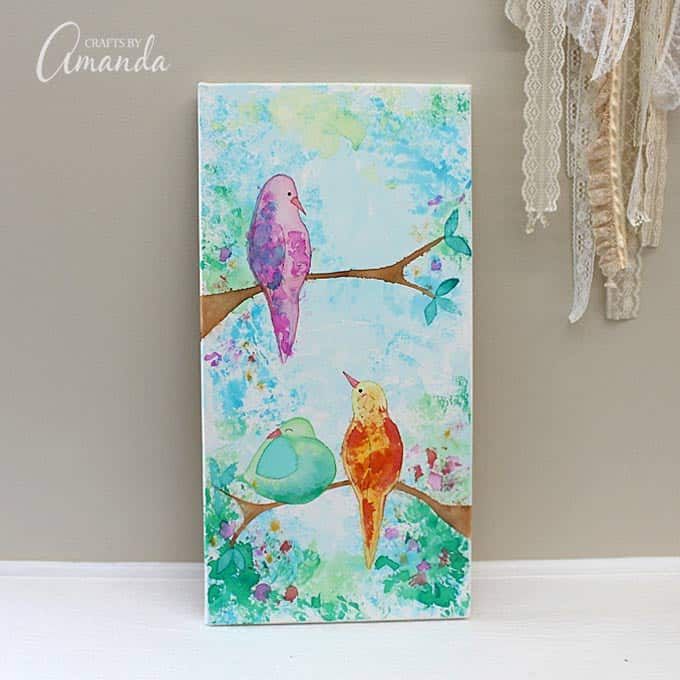In the image, a detailed close-up photograph showcases a rectangular, vertical painting of three whimsical birds perched on two branches, leaning against a beige wall with a white floor beneath. The painting features a playful, abstract background with pastel splotches of green and pink, resembling foliage and flowers. 

On the top branch extending from the left, a purple-pink bird gazes downwards. The bottom branch stretches from the right, supporting a round, light green bird on the left looking towards a brightly colored orange-reddish bird on the right, which in turn looks up at the bird above. A watermark in white text on the top left corner reads "Crafts by Amanda." 

Additionally, in the top right corner of the image, several thin, see-through fabric strings or lacy ribbons in cream tones are artistically draped, adding a touch of delicate texture to the scene.